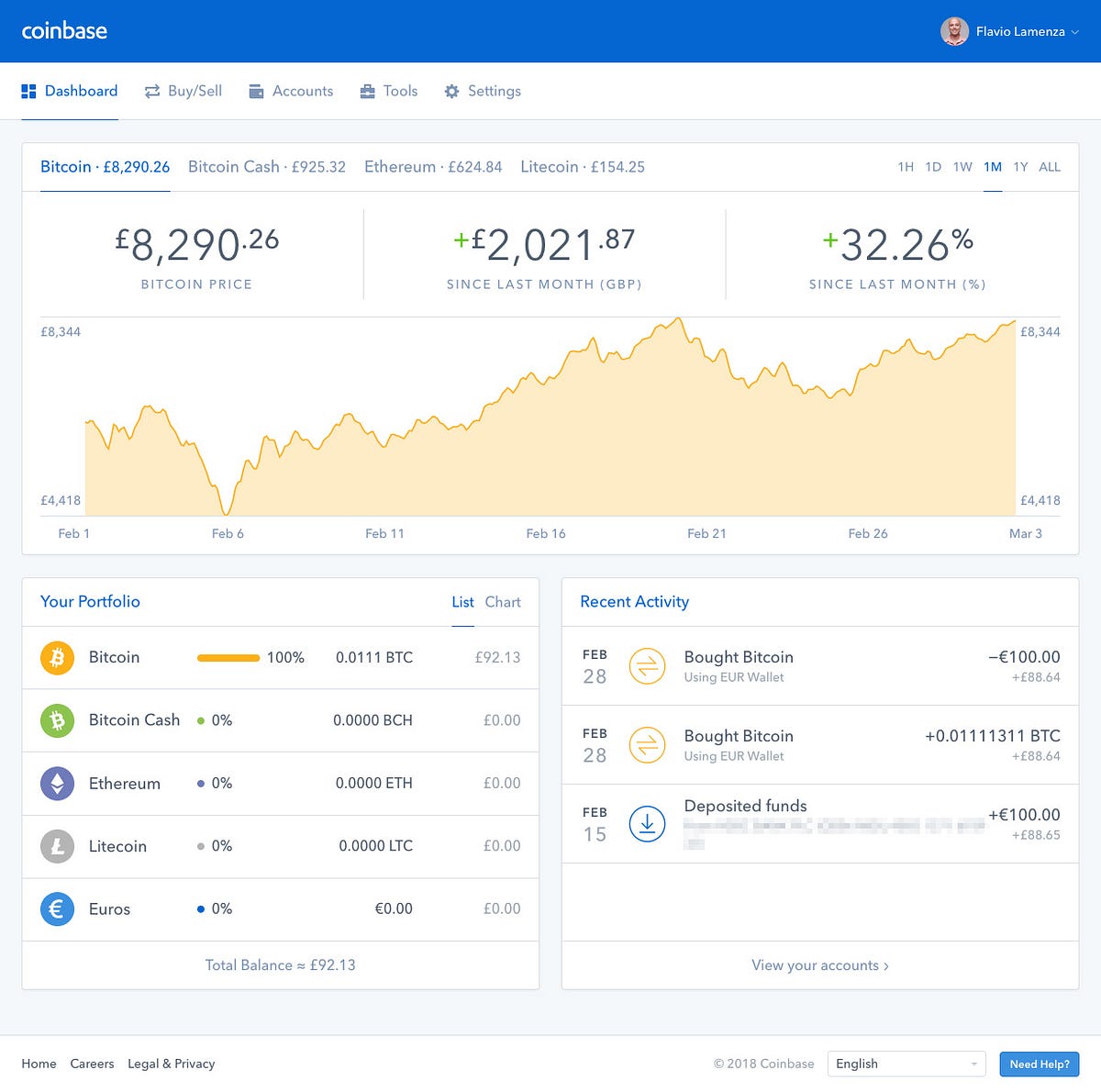Screenshot of a User's Coinbase Holdings in Bitcoin:

At the forefront of this screenshot is the Coinbase interface, distinguished by a blue header bar. In the top-left corner of the header, "coinbase" is displayed in lowercase white letters. On the top-right, the logged-in user's name and profile picture are visible.

Beneath the blue header, a navigation menu is present, showing options: Dashboard, Buy, Sell, Accounts, Tools, and Settings. The Dashboard tab is currently selected.

Dominating the middle section of the screenshot is a large Bitcoin graph. To the top-left of this graph, "Bitcoin" is labeled. Adjacent to this, details of the user's holdings are listed, including Bitcoin, Bitcoin Cash, Ethereum, and Litecoin.

Directly below the holdings summary, the current Bitcoin price is displayed along with comparisons to its value since the previous month, denominated in GBP, and the percentage gain over that period.

The main graph, rendered in red, charts the fluctuations in Bitcoin’s price from February 1st to March 3rd. 

Towards the bottom-left of the interface, a white box labeled "Your Portfolio" enumerates the user's crypto holdings in a vertical list.

On the right side of the screen, a "Recent Activity" section lists three entries detailing the user's recent transactions, specifically the deposits and Bitcoin purchases.